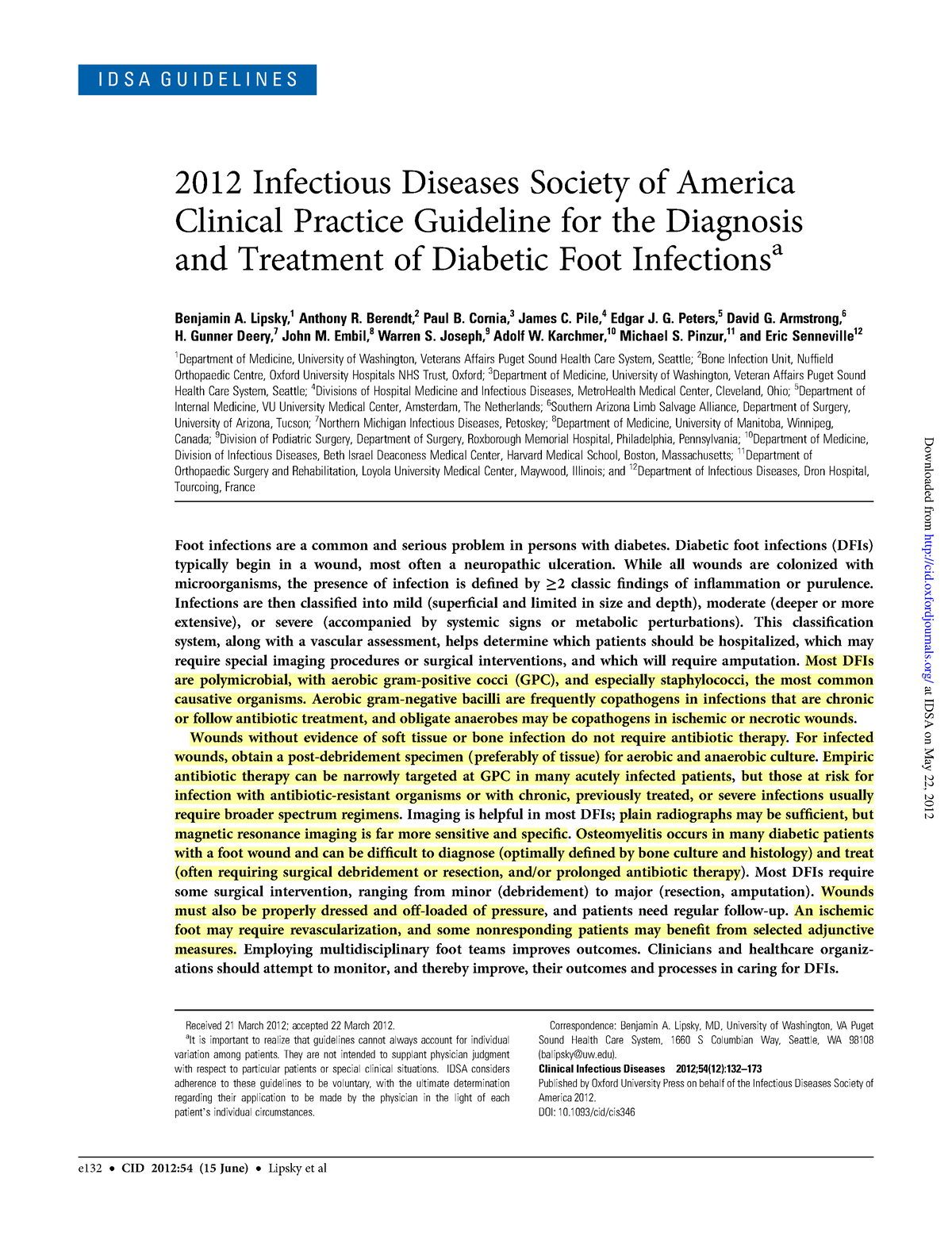A screenshot of an article features prominently at the top-left corner in a blue box, with the text "IDSA Guidelines" displayed in white font. The article is titled "2012 Infectious Disease Society of America Clinical Practice Guideline for the Diagnosis and Treatment of Diabetic Foot Infections." Below the title, a list of contributing authors is presented: Benjamin Lipsky, Anthony R. Barron, Paul Cornea, James C. Pyle, Edgar J.G. Peters, David G. Armstrong, H. Gunnar Deary, John M. Amble, Warren S. Joseph, Adolph W. Cashmere, Michael J. Pinzer, and Eric Senefel. A portion of the article is highlighted, beginning with the information that most diabetic foot infections (DFIs) are poly-microbial, involving aerobic gram-positive cocci, notably indicating a prevalence of these bacteria and their response to antibiotic treatment.